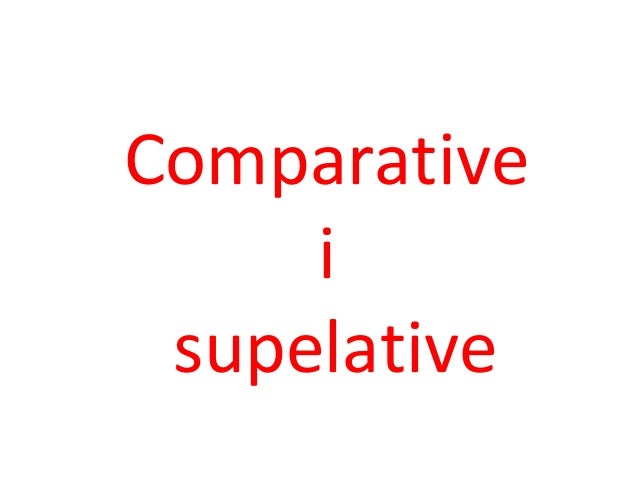The image features a clean, white background with text in large red letters. Centered in the image, "Comparative" is written at the top with an uppercase 'C,' followed by a lowercase 'i' on the next line. Below the 'i,' the word "supletive" appears in all lowercase letters, although it appears to be a misspelling of "superlative," missing the 'r.' The text is well positioned, with each term aligned and spaced evenly, suggesting the style of a title slide from a presentation. This minimalistic design, using only red text against a white backdrop, emphasizes the words and their alignment, potentially playing on the theme of comparison and superlatives.